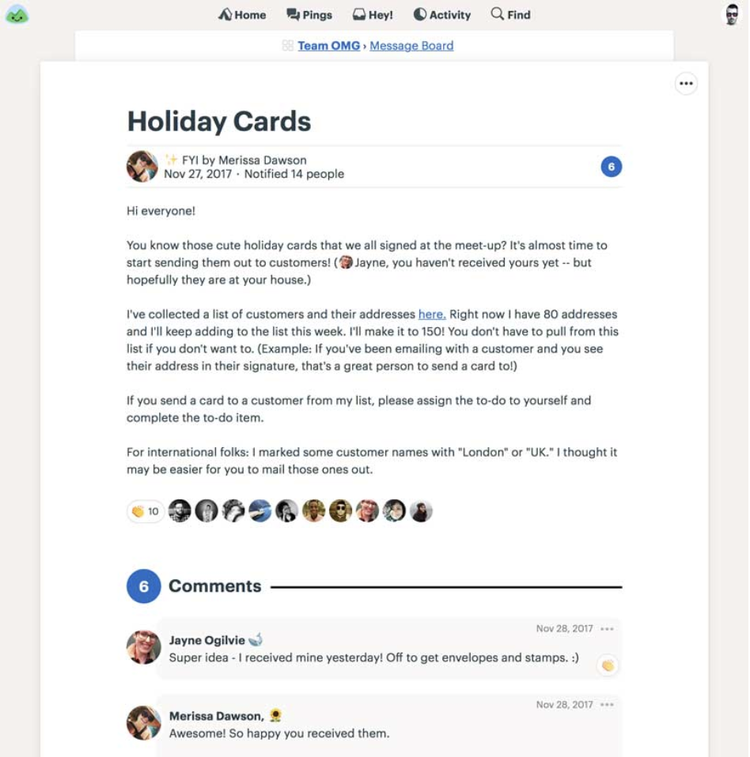**Detailed Caption for Screenshot of TOMG Message Board:**

The screenshot displays a website interface with several navigation icons at the top, labeled: "Home," "Pings," "Hey," "Activity," and "Find." On the main header, it reads "TOMG Message Board" in blue. To the upper left are cartoonish icons, while an illustrated man's head with sunglasses is found to the upper right.

Below the "TOMG Message Board" title, in bold black letters, it says "Holiday Cards." Immediately beneath that, an icon of a picture in brown is followed by the text "FYI by Marissa Dawson," indicating the author and type of post. The date "November 27, 2017," the notification "Notified 14 people," and a blue circled number "6" are also provided in this section.

The body of the message begins with "Hi everyone," and continues to explain that it is time to start sending out the holiday cards that were signed at the meetup. The message indicates that Jane has not yet received hers but should soon. Another paragraph mentions a list of customer addresses which can be accessed via a hyperlink labeled "here" in blue. The text specifies there are currently 80 addresses, with a goal of reaching 150.

The instructions further elaborate that pulling addresses from the list is optional, particularly if you already have customer addresses from prior email signatures. A subsequent paragraph advises assigning and completing a to-do item if sending cards to customers from the list. It also specifies marking some names with "London" or "UK" for international mailing ease.

Beneath this, there's a blue circled number "10" and several circular profile icons of people. Further down, the text "6" in a blue circle and "Comments" in bold black are almost aligned to the right side, with two additional profile pictures appearing below.

One comment from "Jane Ogilvie," dated November 28, 2017, includes a fish icon, expressing excitement about the idea and mentioning she received her cards and is now getting envelopes and stamps. Another response from "Marissa Dawson," dated the same day, features a sunflower icon, confirming her happiness that Jane received the cards.

This comprehensive message details the holiday card sending effort, customer address organization, and updates from team members.